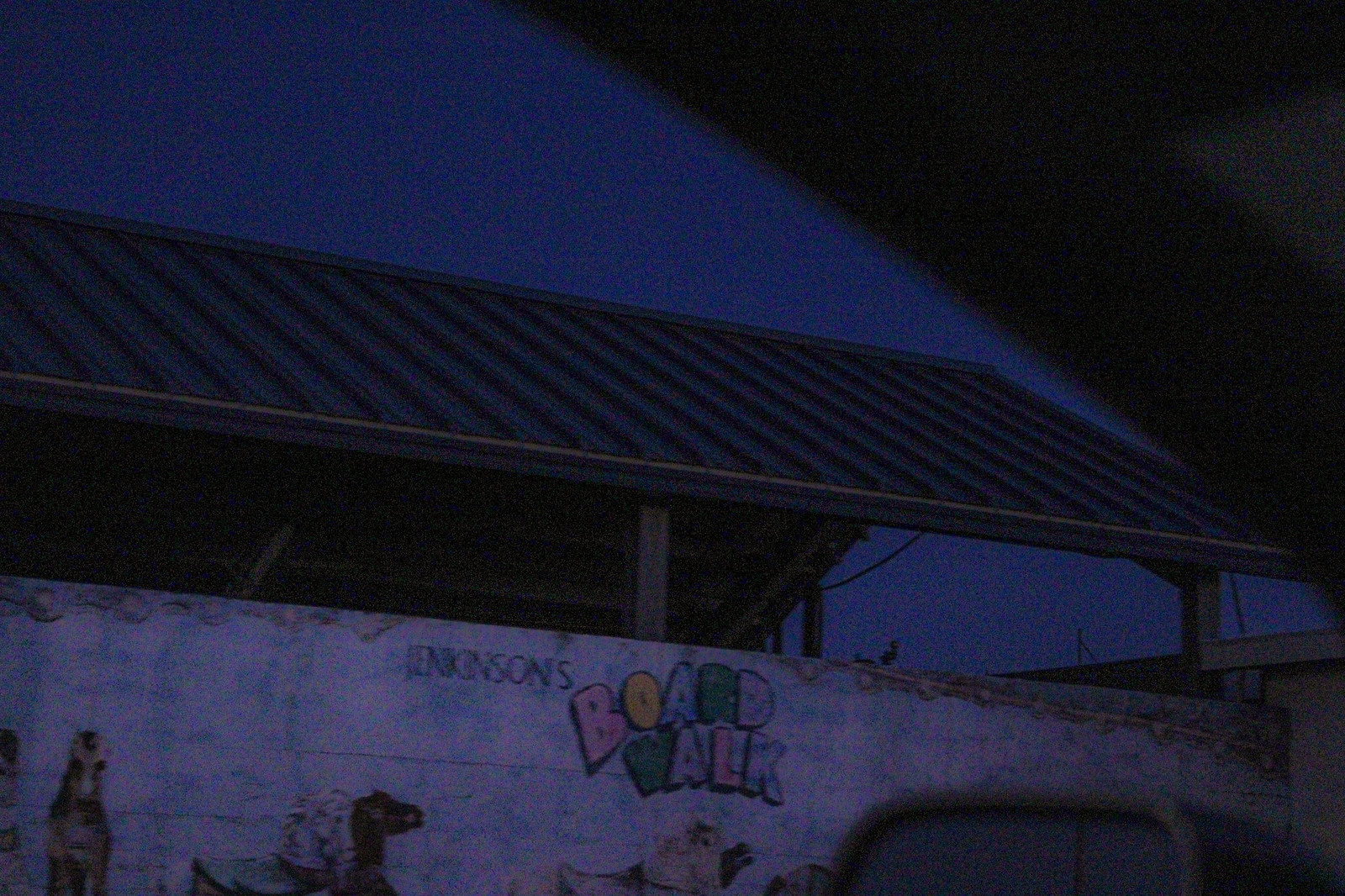The image is a dark, nighttime photo taken from the driver's side window of a car, capturing a white concrete wall adorned with graffiti. The prominent text, which reads "Nickinson's Boardwalk," is painted in black for "Nickinson's" and in colorful bubble letters—pink, yellow, blue, and green—for "Boardwalk," arranged in a jaunty slant. The wall also features painted animals; among them, a dinosaur and a horse are discernible on the bottom left. In the bottom right of the image, part of the driver's side rear view mirror is visible, while the top right shows a portion of the door frame. The scene includes a metal roof, supported by wooden poles, that appears to shelter an open area behind the wall. The image has a dim, bluish cast, enhancing the slightly mysterious and urban nighttime atmosphere.